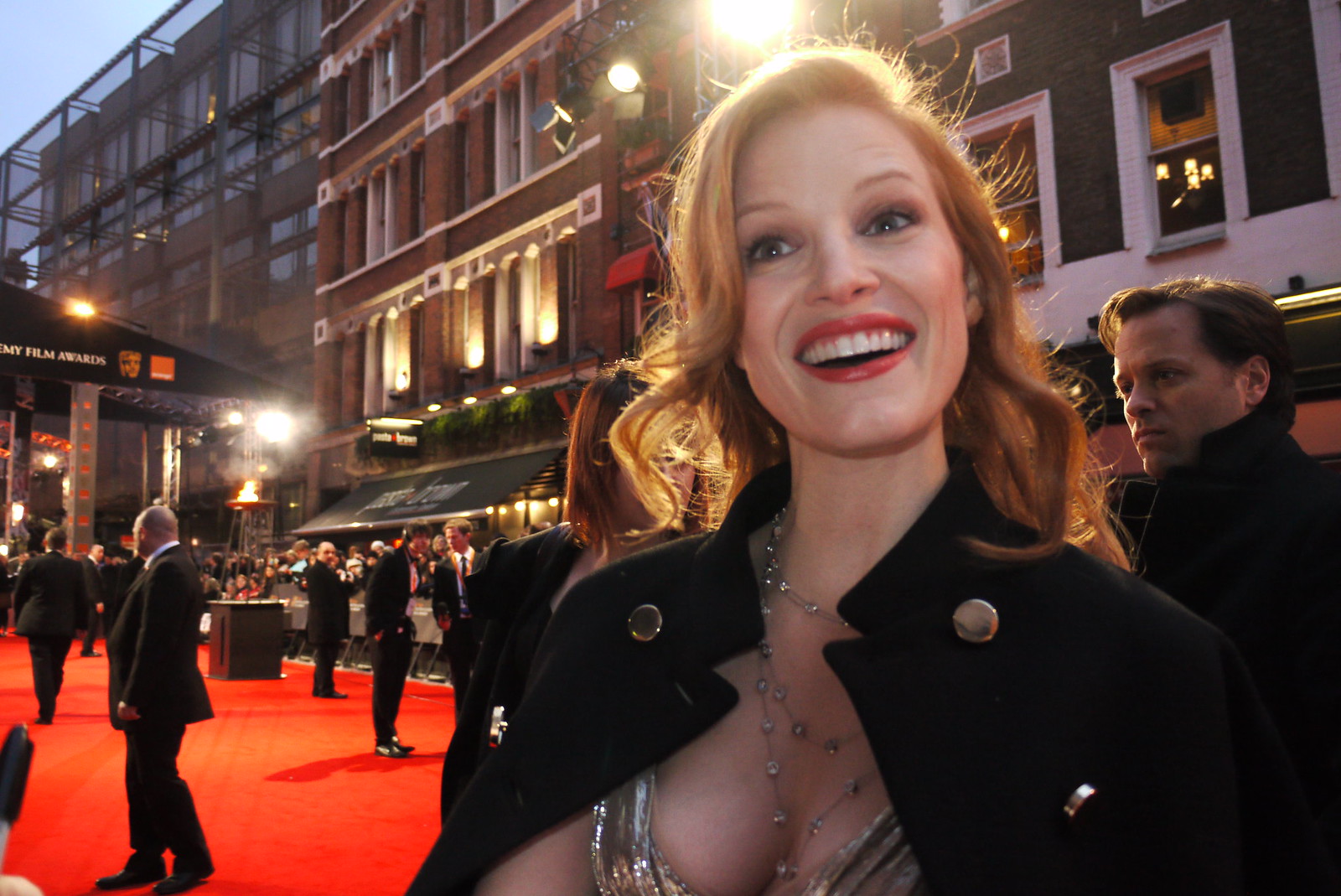In this outdoor image, an elegant event is taking place. The scene is set on a city block featuring a row of multi-story buildings, one of which has a substantial, light-adorned awning on the left side, supported by large beams. The vibrant red carpet stretches across the entire street in front of these buildings, denoting a special occasion. Various individuals, primarily dressed in black suits, are seen standing on the carpet and nearby sidewalks, with some chairs arranged in front of one of the buildings.

At the focal point and center of the image is a vivacious woman with wavy red hair cascading to her shoulders. She is finished to perfection with makeup, highlighted by bright red lipstick and a radiant smile. Her ensemble includes a standout black coat with large gold buttons flanking each side of the collar, a stunning, sparkling silver dress with a low-cut neckline, and an array of jewels adorning her neck. This image, captured with clear skies and daylight, showcases a well-dressed crowd amidst a sophisticated, urban backdrop, creating a lively and refined atmosphere.